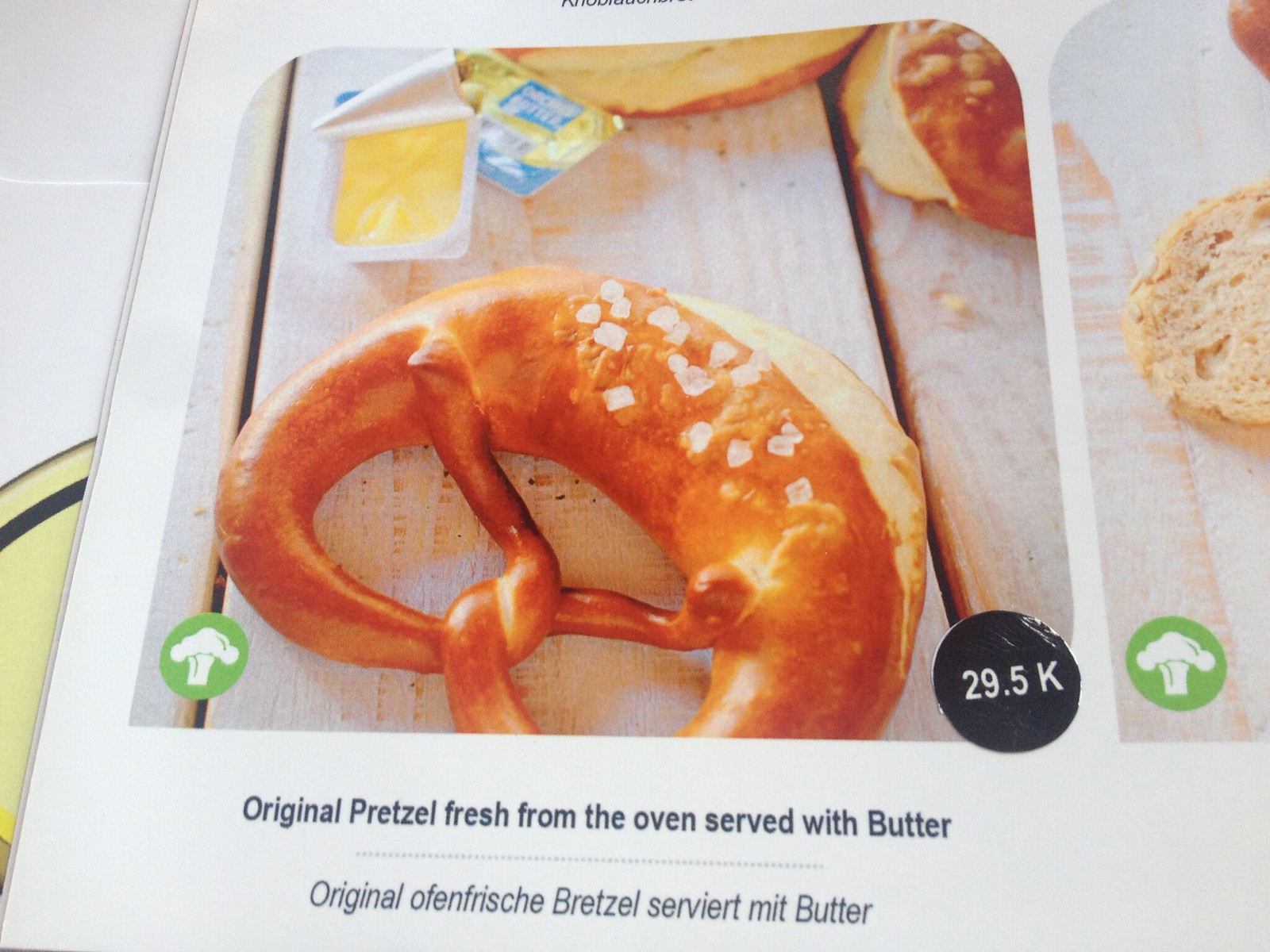The image features a detailed photo of a large, lightly browned pretzel with a thick bottom, prominently displayed on what appears to be a white laminate menu or magazine page. The pretzel is generously sprinkled with chunky grains of salt. Beside it, there are two small plastic containers of butter, one with its foil lid peeled back to reveal the yellow butter inside, suggesting it's ready to be spread on the pretzel. In the background, partial views of other pretzels or bagels are visible, though not featured as prominently. To the bottom left of the image, there is a green circle with a white broccoli illustration, likely indicating that the pretzel is vegetarian-friendly. On the bottom right, a black circular sticker bears the text "29.5 K" in white. Below the photo, the caption reads in black text: "Original pretzel, fresh from the oven, served with butter," followed by a translated version, possibly in German.